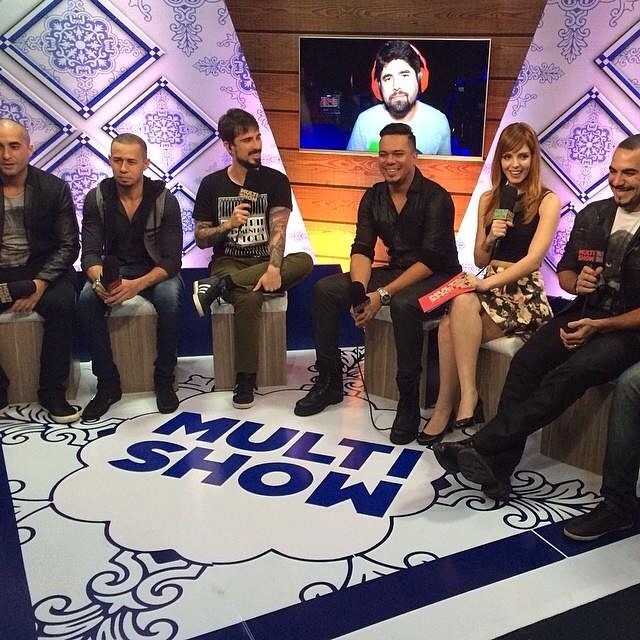The image depicts a lively talk show set, featuring six individuals seated on backless stools with white cushions and brown bases. Each person, dressed predominantly in black attire, is holding a microphone with a black top. One female panelist, positioned second from the right, stands out with her long red hair, black sleeveless tank top, black floral skirt, and heels, holding a set of orange cards. She appears ready to lead the discussion. Behind her, a TV monitor displays a man wearing red headphones and a white shirt. The stage is adorned with a blue diamond-patterned wall and a matching floor design, creating a cohesive backdrop. At the center of the floor, large blue letters spell out "multi-show," marking the theme of the event.